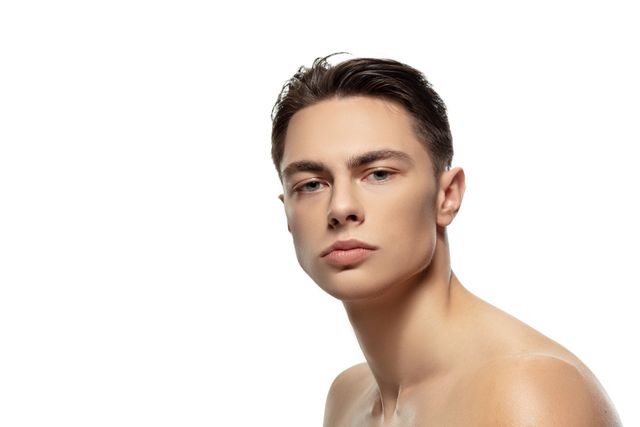A full-color, high-resolution photograph captures a young Caucasian male, likely in his 20s, set against a stark white background with no border or additional text. The man, who has short, dark hair meticulously combed back and slightly spiky in the front, presents a clean-shaven, well-groomed appearance. He is shirtless, revealing his bare shoulders and the entirety of his left ear, with just a portion of his right ear visible. His piercing blue eyes, framed by thick eyebrows, gaze directly into the camera with a neutral, almost introspective expression. His left shoulder is angled towards the camera, giving the impression of looking over it, enhancing the photo’s dynamic composition and emphasizing the subject's contemplative mood. The plain, white backdrop underscores the focus on his striking features and well-maintained look, subtly suggesting he might have just stepped out of the shower.